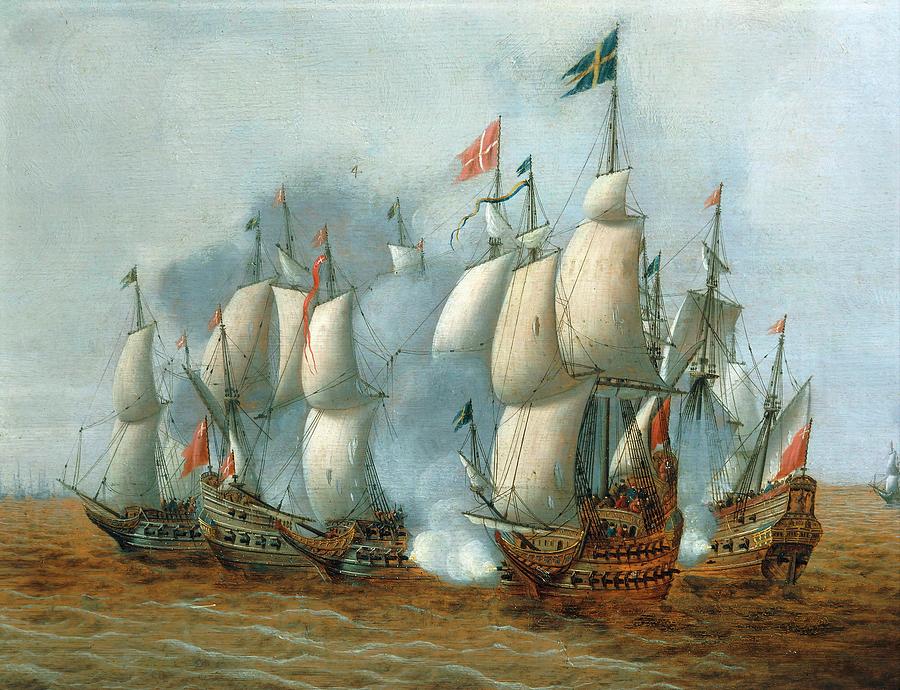A vibrant painting depicts a dramatic naval battle from the colonial era, with five or six grand wooden warships engaged in fierce combat on a turbulent sea. The ships, with towering three-masted structures and large billowing white sails, are positioned strategically, broadside to one another, firing rows of cannons that emit thick clouds of smoke. Each vessel is adorned with a distinct flag at the top of its masts, including a blue flag with a gold cross and a red flag with a gold cross, symbolizing their different countries of origin. The sea beneath them has a brownish hue with specks of blue, suggesting churning waters amid the conflict. The background features a partly cloudy blue sky, enhancing the chaos and grandeur of the scene. The meticulous details capture the intensity of the moment, from the wind-filled sails to the ensigns fluttering in the breeze, conveying the historic essence of maritime warfare.